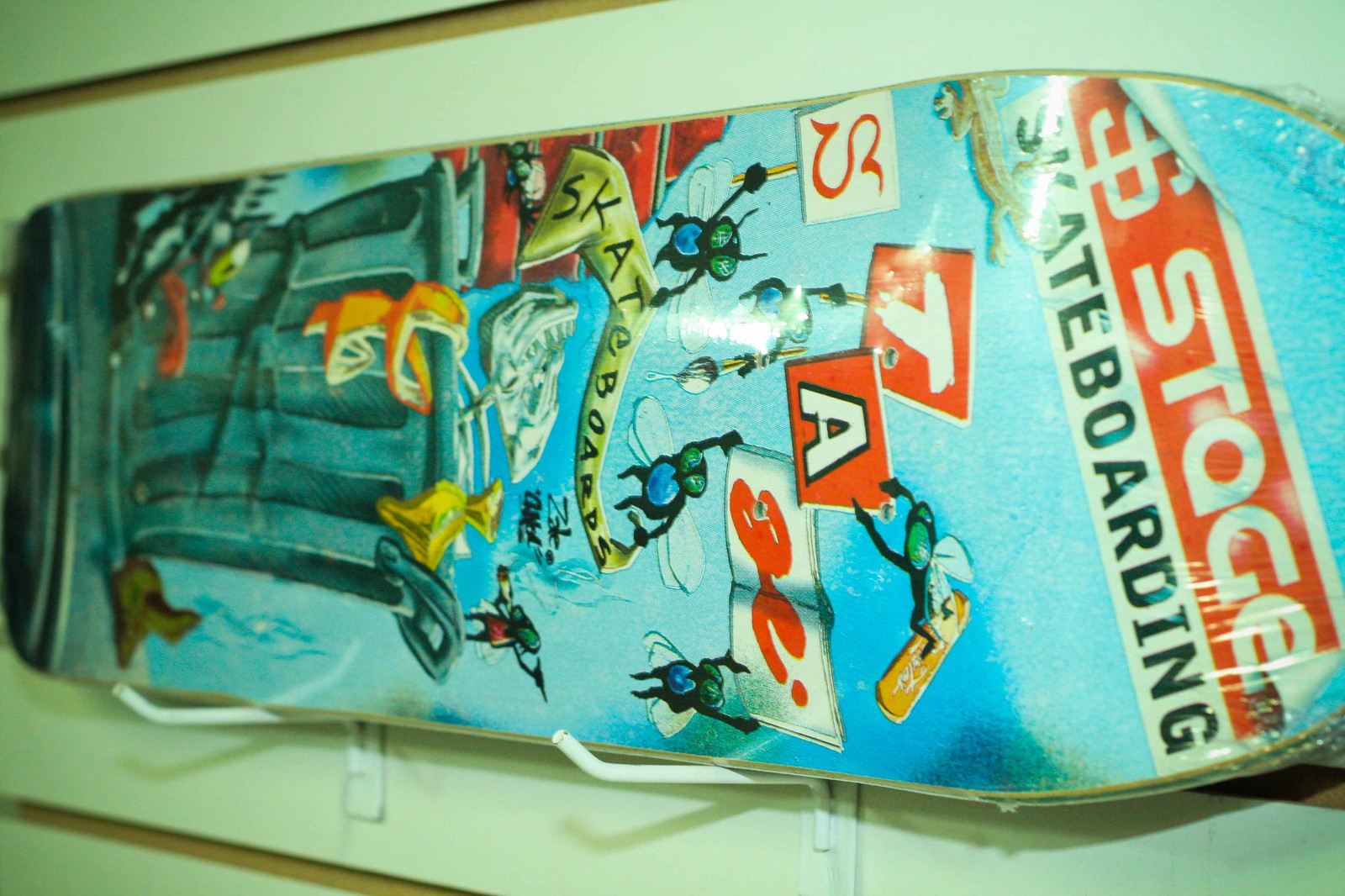This is a color photograph of a skateboard deck affixed to a wall in a horizontal position, resting on two white brackets against horizontal white planks. The skateboard, which lacks wheels, has its tail facing the left edge of the image and its cropped nose pointing to the right. The bottom of the deck features detailed, painted graphics on a blue background. At the top, a red banner with a peeling corner displays a dollar sign followed by the word "STAGE" in white lettering. Beneath this is a white rectangular box with the word "skateboarding" in black text. Below, several black and blue flies are depicted in various poses around the letters S, T, A, G, and E, which are presented in different type fonts. Some flies hold the letters, while others are shown skating or interacting with a trash can that has several trash pieces scattered around it. The imagery combines elements of computer graphics and photographic representationalism realism.